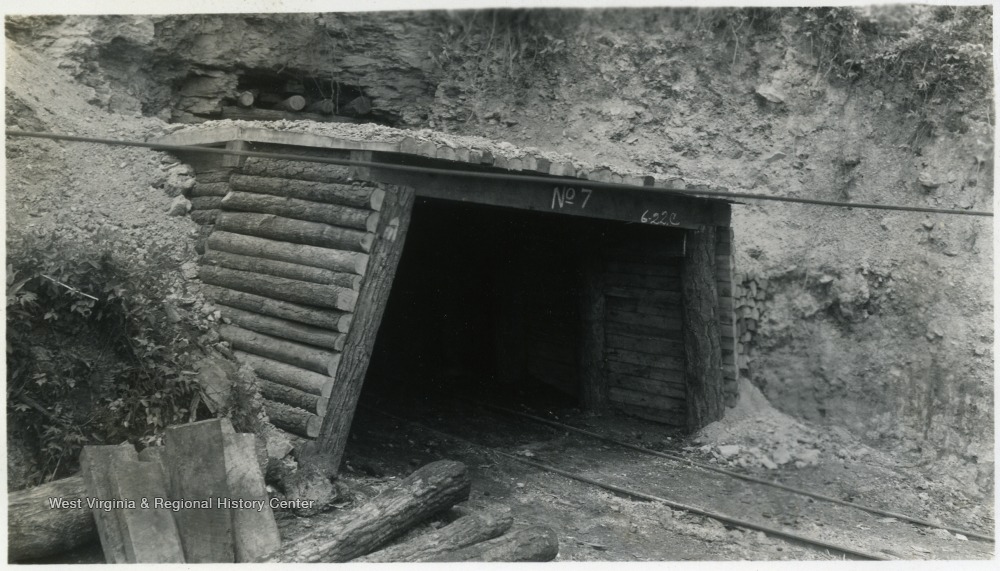The black-and-white image appears to be an historical photograph depicting the entrance to an old mine. The mine's entrance is framed by a wooden archway constructed from halved logs, giving it a rustic, sturdy look. A set of tracks, likely for mine carts, runs into the dark opening of the mine, set amidst a large, excavated dirt hill. Above the entrance, there are markings, notably "No. 7" and "6-22.C," indicating either a mine shaft number or some form of identification. In the lower left of the image, a neat pile of logs or lumber can be seen, and a wire horizontally spans the scene above the archway. The setting is bathed in natural light, making the details of the scene clear despite its monochromatic portrayal. In small white writing at the bottom left corner, the text reads "West Virginia and Regional History Center," signifying the image's archival source. The overall scene is devoid of people or vehicles, offering a stark yet detailed glimpse into a piece of industrial history.